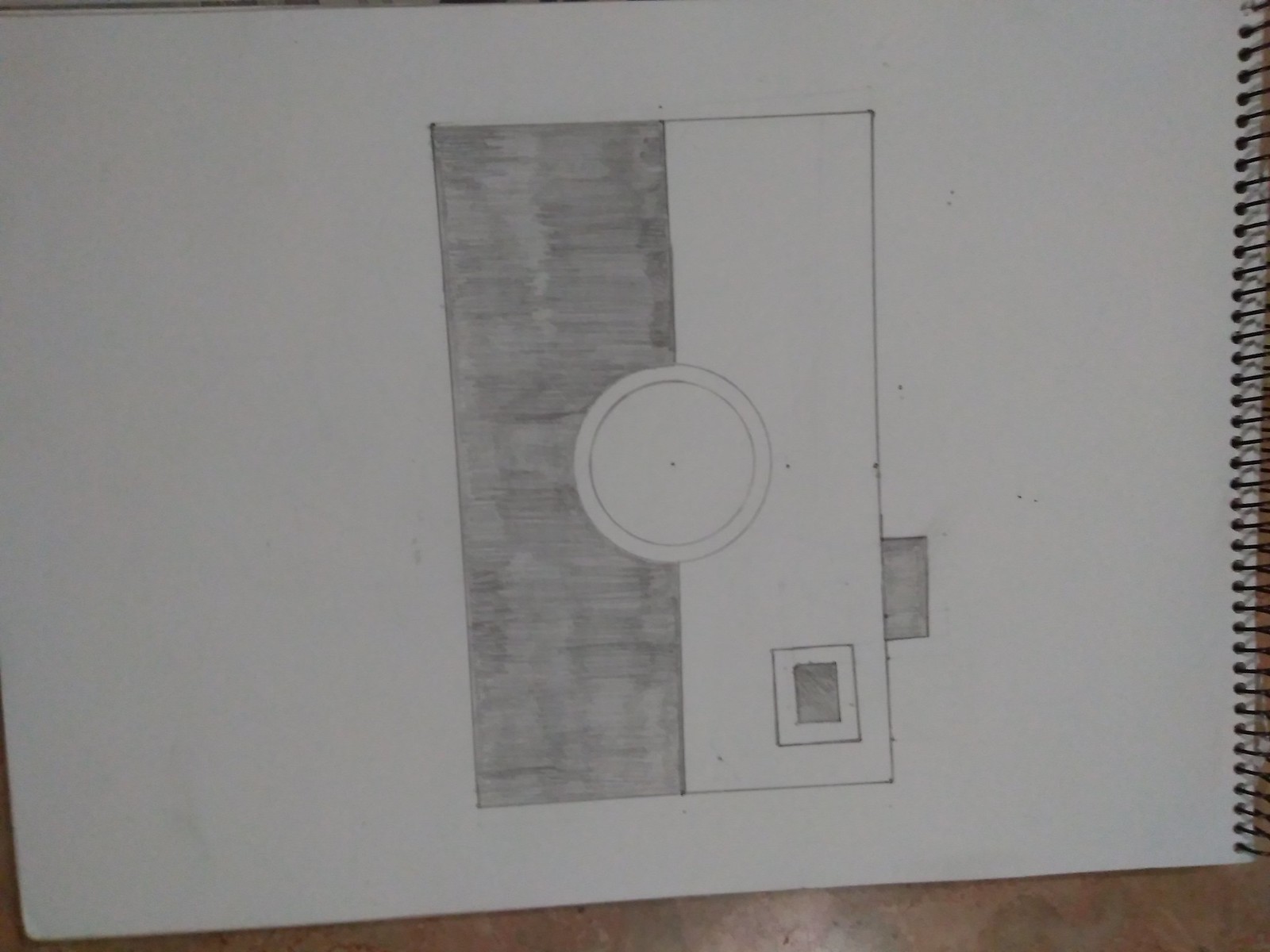This photograph captures a pencil sketch rendered on a large, white sheet of paper within a spiral-bound notebook. The notebook's black spiral binding is visible along one edge, contributing to a slightly blurred composition that hints at the image's vintage nature. The sketched object is a point-and-click camera, depicted in a vertical orientation suggestive of the camera being turned. Central to the sketch is a circular lens, meticulously placed to bring focus to the camera's face. The lower portion of the camera is shaded black to contrast with the upper part, which remains white, creating a stark division. Notably, a black-shaded button is illustrated at the camera's top, signifying the shutter button typically pressed to capture a photo. Adjacent to this button, the viewfinder and flash are represented as a square feature; part of this square is shaded in black while the remaining section is left white, enhancing the sketch's monochromatic aesthetic.